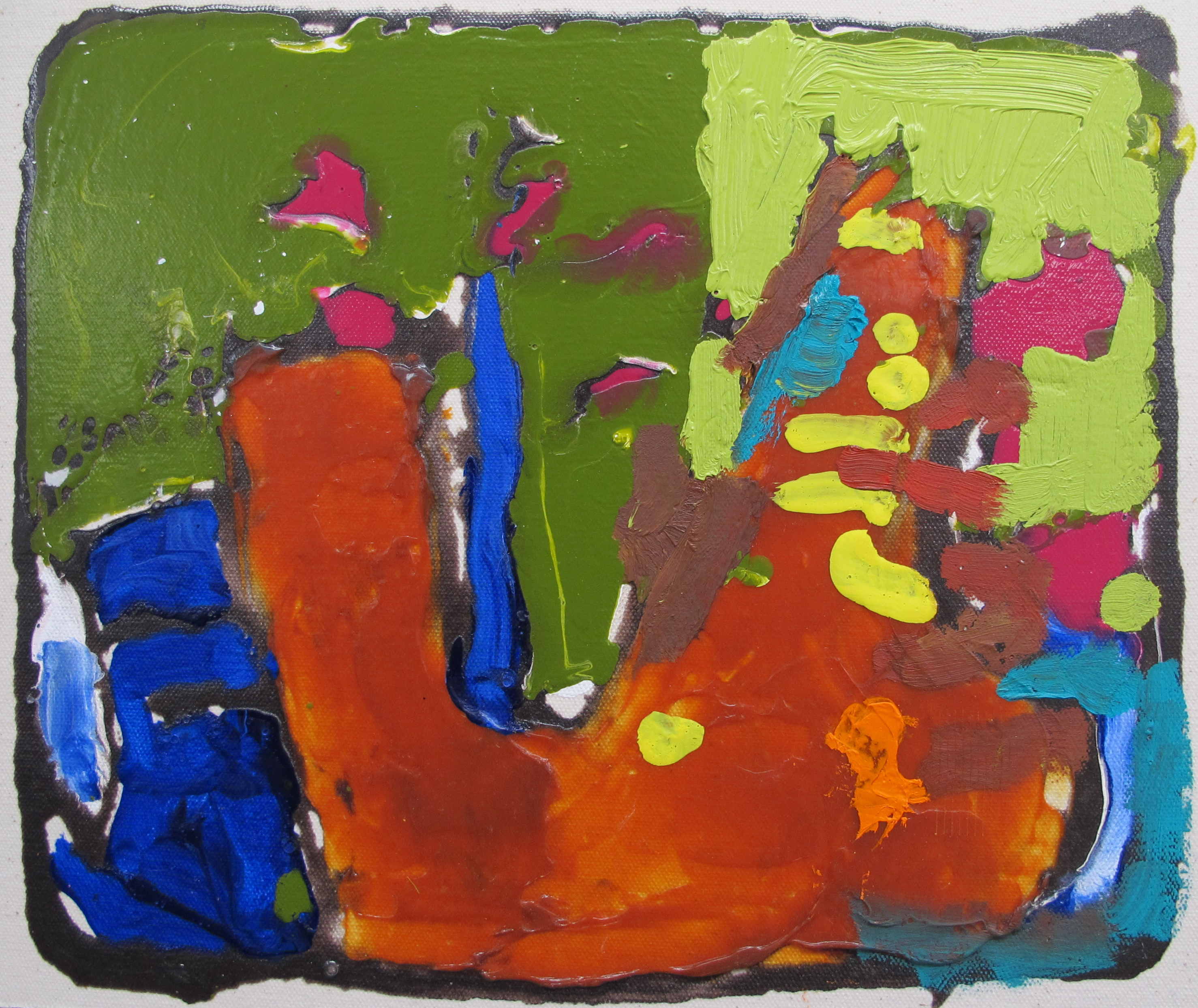This painting appears to be an abstract piece with a childlike quality, featuring a chaotic and seemingly haphazard blend of bright, bold colors and shapes. The background is a wide vertical rectangle with a gray hue, bordered by a dark gray frame that transitions into black on the lower half. Dominating the composition is a large, deep orange U-shaped figure with an appendage on the side, which stands out against the mixed backdrop.

In the upper left corner, there is an area of dark, avocado-like green, interspersed with bright blues and small patches of white. The upper right corner hosts a lime green section surrounding part of the U-shape, accented with pink blotches. Toward the lower right, shades of teal and black meld together with blue streaks, creating a sense of depth and texture.

Further adding to the vibrant ensemble, yellow and white dots are scattered throughout the painting, joining various shades of pink, dark blue, and other hues. This medley of colors and forms evokes a sense of spontaneous creativity, akin to a finger painting or a collage where the paint appears to flow and blend into itself, resulting in a vivid and lively abstract artwork.